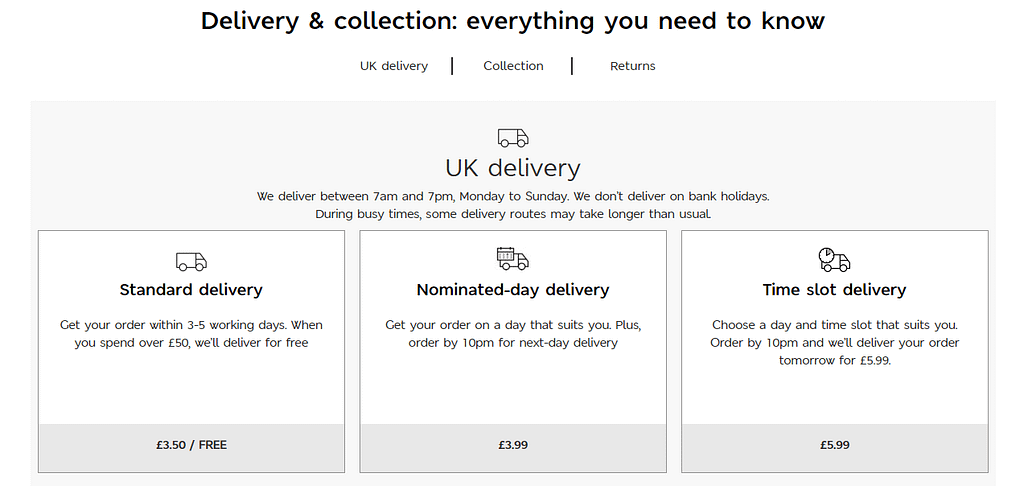**Descriptive Caption:**

The image is a detailed screenshot from an unidentified UK-based website, focusing exclusively on delivery options and logistics. The webpage has a minimalist design with a predominantly white and gray background juxtaposed with black text. The only visual elements are a few cartoonish truck icons denoting different delivery methods and their associated costs.

The screenshot is headed by the title "Delivery and Collection: Everything You Need to Know." It then lists three main options: UK Delivery, Collection, and Returns, indicating a European origin—explicitly the UK, inferred from the currency used and terminology.

The chosen section is UK Delivery, detailing service times and exclusions. Deliveries are made between 7 a.m. and 7 p.m., Monday through Sunday, excluding bank holidays. There's a note mentioning potential delays during peak periods. Three delivery options are available:

1. **Standard Delivery:** The most economical choice.
2. **Nominated Day Delivery:** A mid-tier option allowing the customer to select a preferred delivery date.
3. **Time Slot Delivery:** The premium, most expensive option, offering a precise delivery window.

This clear, methodically cropped portion of the webpage aims to provide essential delivery information in a straightforward, user-friendly manner.